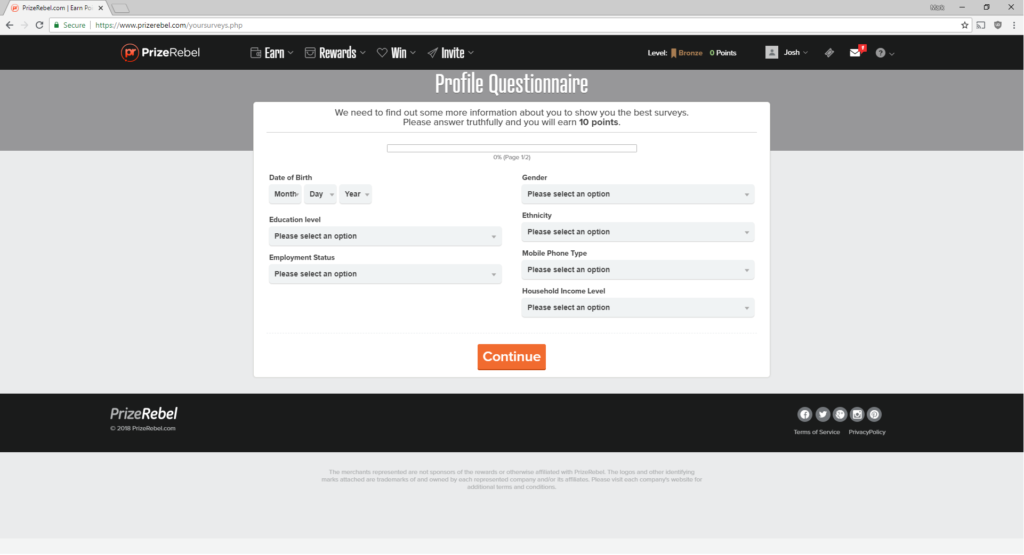This is a detailed screenshot of the PrizeRebel.com website, showcasing a pop-up box titled "Profile Questionnaire." The pop-up requests additional user information to personalize survey options, promising a reward of 10 points for truthful answers. Users are prompted to input data through options including Date of Birth, Education Level, Employment Status, Gender, Ethnicity, Mobile Phone Type, and Household Income Level, each accessible via drop-down menus. At the bottom of the questionnaire, an orange "Continue" button is prominently displayed. 

The website's main interface is primarily black, white, and gray, offering a clean and minimalistic design, with accents of color for emphasis. The PrizeRebel logo, featuring the letters "PR," is highlighted in a reddish-orange hue. In the upper region of the screenshot, a level indicator shows the user’s status as "Bronze," depicted in a light orange shade. The account's point balance is displayed as "0," numbered in green. Adjacent to these details, there is a square icon with a generic silhouette labeled "Josh" and a message button marked with a small red box indicating one unread message.